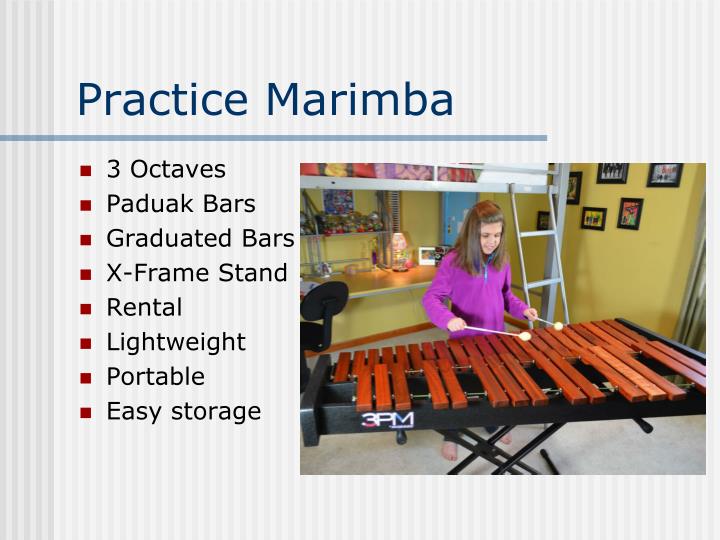In the image, a young girl with shoulder-length brown hair is playing a modern-style marimba, which is similar to a xylophone but involves striking with drumsticks. She is positioned on the right side of the frame and is holding sticks with oval-shaped ends. The marimba has a sleek black and brown frame and sits on an X-frame stand. The instrument, branded "3 p.m.," features graduated padauk bars spanning three octaves. The girl is dressed in a purple jacket and dark trousers, and she is barefoot. The setting is a room with yellow walls adorned with pictures framed in black and a gray-framed bunk bed in the background. The text above the image reads "practice marimba," and on the left side of the image, it lists features of the marimba: "three octaves, padauk bars, graduated bars, x-frame stand, rental, lightweight, portable, and easy storage." The overall design of the image resembles an amateurish ad, with a somewhat cheesy graphic layout and an unappealing choice of colors and fonts.